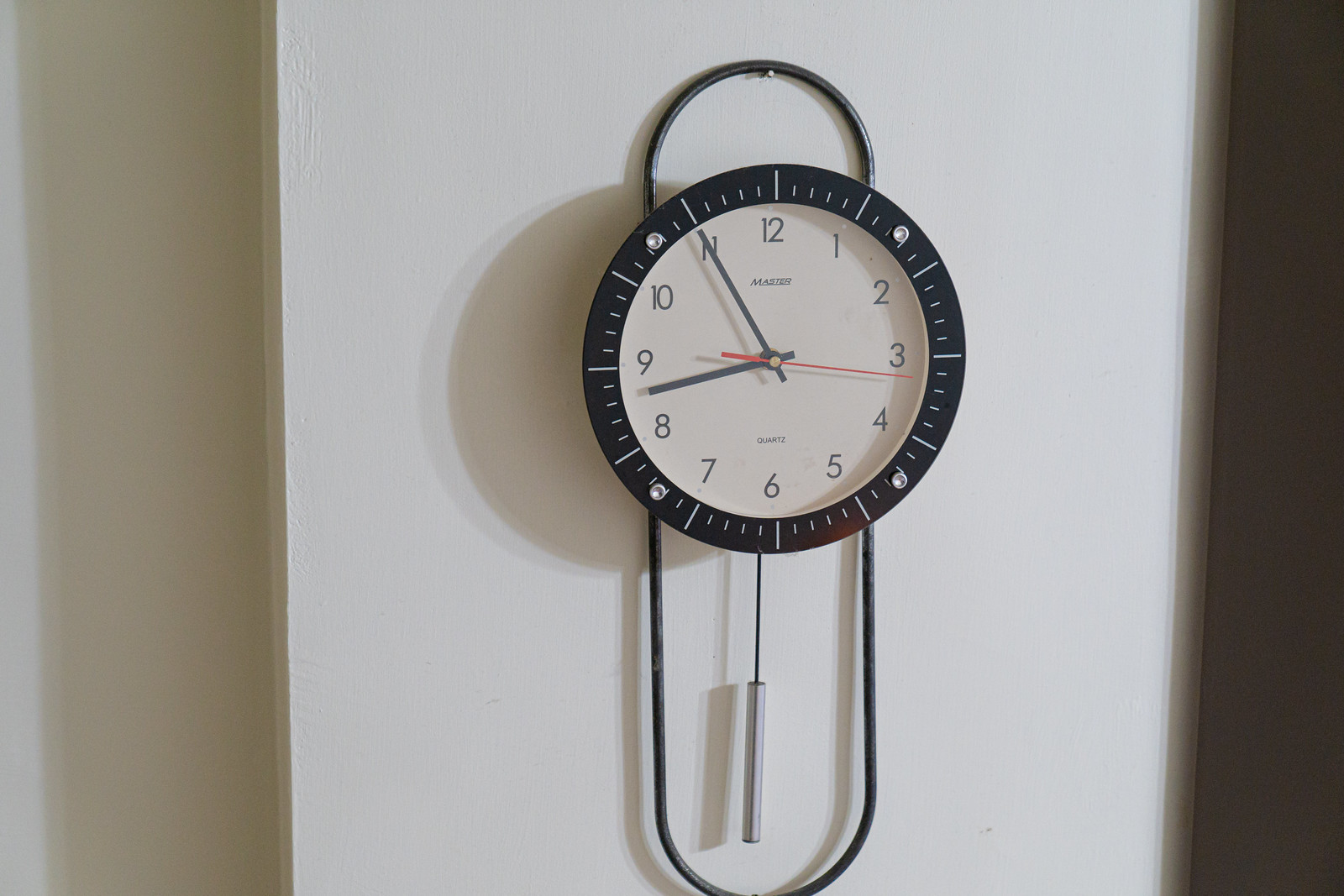This photograph captures a clock hanging on a plain white wall. The clock has a round face with a broad black rim, on which minute markings are painted, and a white interior featuring black numbers. It shows the time as around 8:55, with the black hour and minute hands positioned just below the nine and on the eleven, respectively, and a red second hand pointing at the three. The timepiece also includes a silver pendulum swinging below its oval-shaped, vertically oriented iron base. The clock is suspended by a wire attached to a nail, extending about two and a half times the clock’s length. The wall casts shadows both to the left and right of the clock, with a dark line visible to the right side of the photograph.